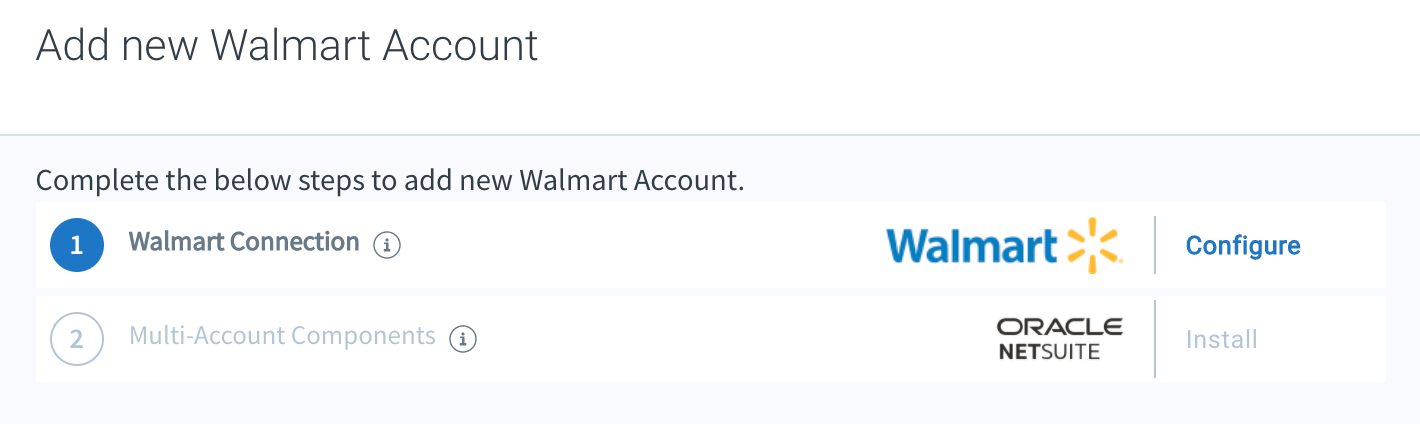The image from the Walmart website displays the "Add New Walmart Account" page prominently on the left-hand side against a light blue background. At the top left, the text "Add New Walmart Account" is written in a larger, thin black font. Below this heading, the page instructs users to "complete the below steps to add new Walmart account." 

The instructional steps are highlighted with numbered indicators:
1. The first step, labeled "Walmart connection," is emphasized within a blue circle with a white number "1."
2. Beneath this, the second step is labeled "multi-account component" and is displayed in a light gray font with a gray number "2" preceding it.

The upper right-hand side of the image is blank, providing a clean contrast to the detailed content on the left.